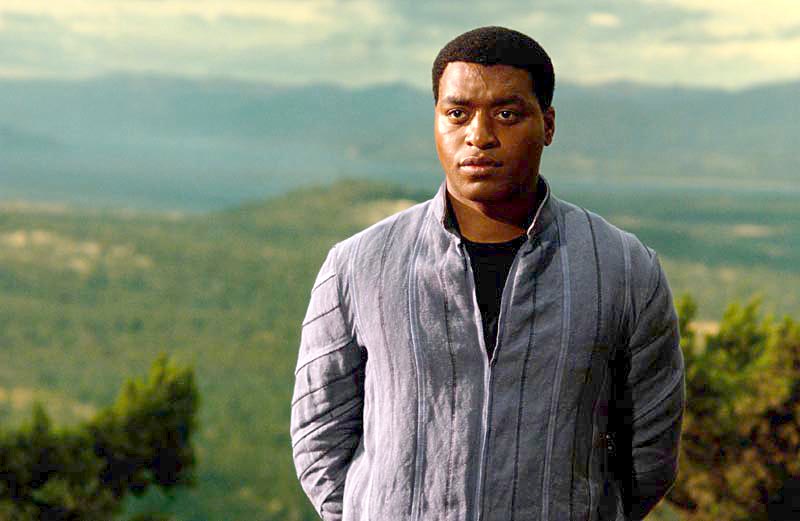In this image, we see a detailed outdoor setting, presumably taken during the middle of the day. The foreground features a large, mostly grassy area with some bushes and trees scattered about. In the distance, there are mountain ranges, and above them, a sky partially covered with clouds. The colors present include light blue, white, gray, dark blue, green, tan, brown, and black, giving the image a natural and serene look.

At the center of the image, slightly to the right, stands an African-American male. He is in sharp focus, while the background remains blurred, drawing attention to him. The man has short black hair and is wearing a gray jacket with vertical stripes underneath, paired with a black t-shirt. His arms appear to be behind him, and the frame cuts off at his stomach. He seems to be looking slightly to the left, not directly at the camera.

The overall setting suggests a vast, open field with prairie-like land and large hills or mountains in the far background. The man, possibly a familiar figure in entertainment, stands out against the natural backdrop, creating a striking and balanced composition.